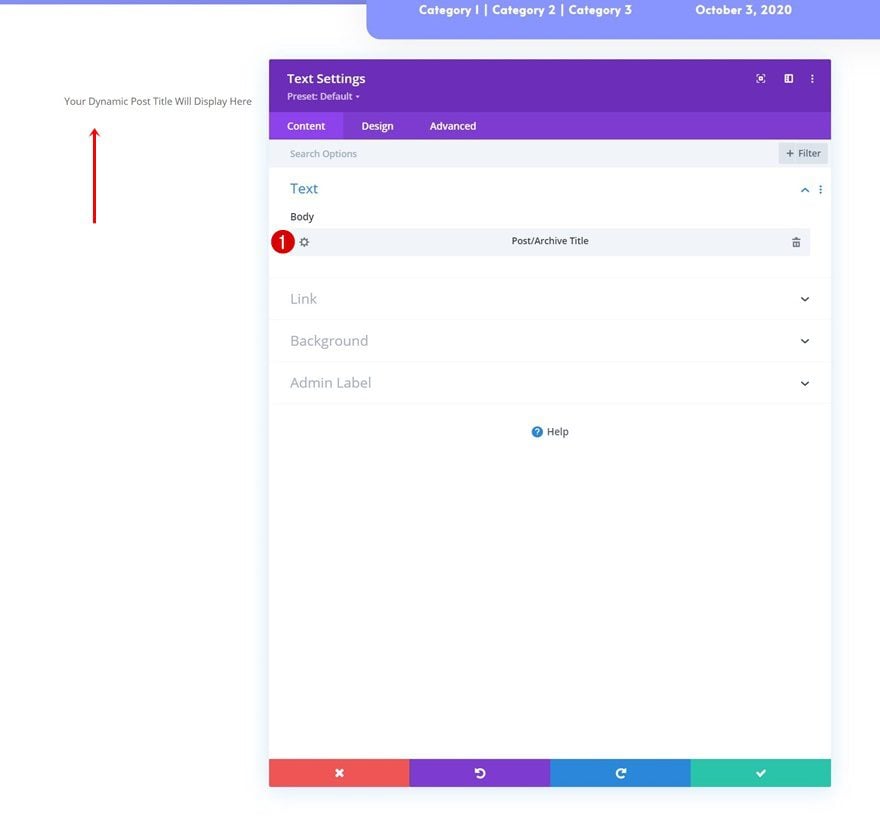The image features a webpage interface mockup in a square format. The background is predominantly white with no visible borders. Across the top, a medium blue line with a pastel tone stretches horizontally. On the right side of this line, a light blue rectangular section with curved edges contains the white text "Category 1," "Category 2," and "Category 3," separated by vertical lines. Near the upper right corner, the text "October 3, 2020" is displayed.

Below this, the primary portion of the image reveals a webpage layout with a white background. The header is purple. At the bottom, four pastel-colored sections sit side by side in orange, purple, blue, and green. The orange section features a white "X," the purple section has a rewind icon, the blue section shows a fast-forward icon, and the green section contains a check mark.

In the upper left of the purple header, "Text Settings" is displayed, followed by “Preset Default” and a downward arrowhead icon. Below this are three clickable sections labeled "Content," "Design," and "Advanced," with "Content" being highlighted.

In the main white section, the upper left reads "Text" with "Body" below it. A red circle with a white number "1" appears beneath "Body," accompanied by a gears icon to the right in a long gray bar that reads "Post/Archive Title." Further down are sections labeled "Link," "Background," and "Admin Label," with downward-facing arrows to the right for expanding options. Centered beneath “Admin Label” is a blue circle with a white question mark labeled "Help."

Outside this main white area, to the left, is an upward-facing red arrow. Above this arrow, in small gray text, it reads, "Your Dynamic Post Title Will Display Here."